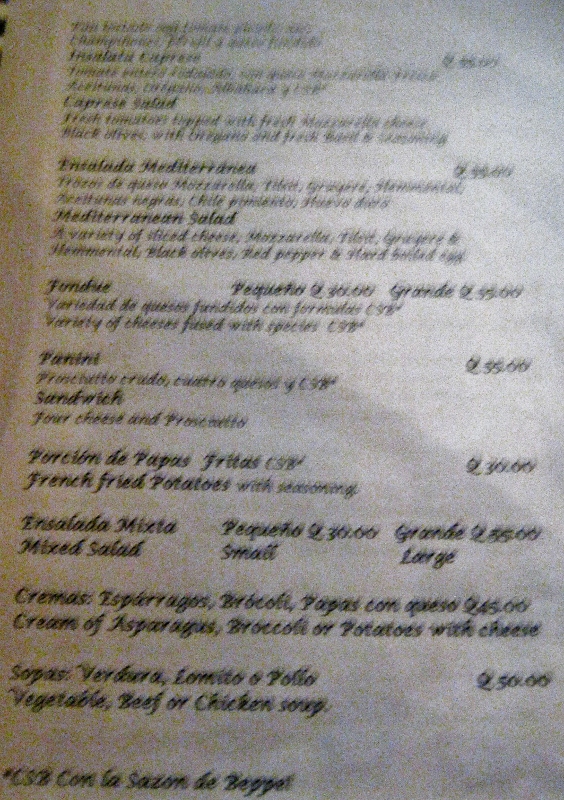This photograph shows a severely out-of-focus menu set against a white background with black text. The blurred top half of the menu renders it unreadable, but a closer look at the lower half reveals several menu items listed in both English and Spanish, though some descriptions remain indecipherable due to the smaller font size. The first legible line is “Caprese Salad,” followed by “Ensalada Mediterranea” and its English equivalent, “Mediterranean Salad.” Other items on the menu include “Fondue” listed at a price of 55 (currency unclear), “Panini,” “Sandwich,” “Four Cheese and Prosciutto,” and “French Fried Potatoes.” Two versions of salad are available: “Ensalada Mixta” or “Mixed Salad,” which come in small or large portions. Soups listed include “Cream of Asparagus,” “Broccoli or Potatoes with Cheese,” and “Vegetables, Beef or Chicken Soup.” The prices for these items range between 30 and 55 units of an unspecified currency.